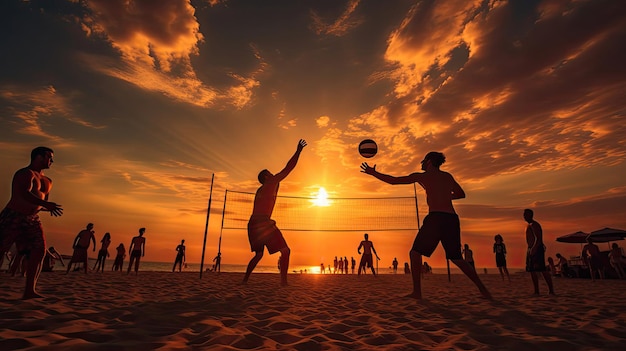In this captivating sunset beach scene, a lively volleyball game unfolds as the sun dips towards the horizon, casting a glowing orange and yellow hue across the sky, intermixed with deep blues and purples. The photograph, taken from a low angle, gives the viewer an immersive perspective, making it feel as if they are amidst the action. In the foreground, two players stretch towards a volleyball suspended mid-air above the net. Their muscles tense in anticipation, as other beachgoers and players populate the scene, some gathered under umbrellas on the right, enjoying the mellow evening atmosphere. The water in the background glistens with the sun's reflection, and the clouds scattered across the sky add depth to this picturesque moment, almost appearing like they are chasing the descending sun.